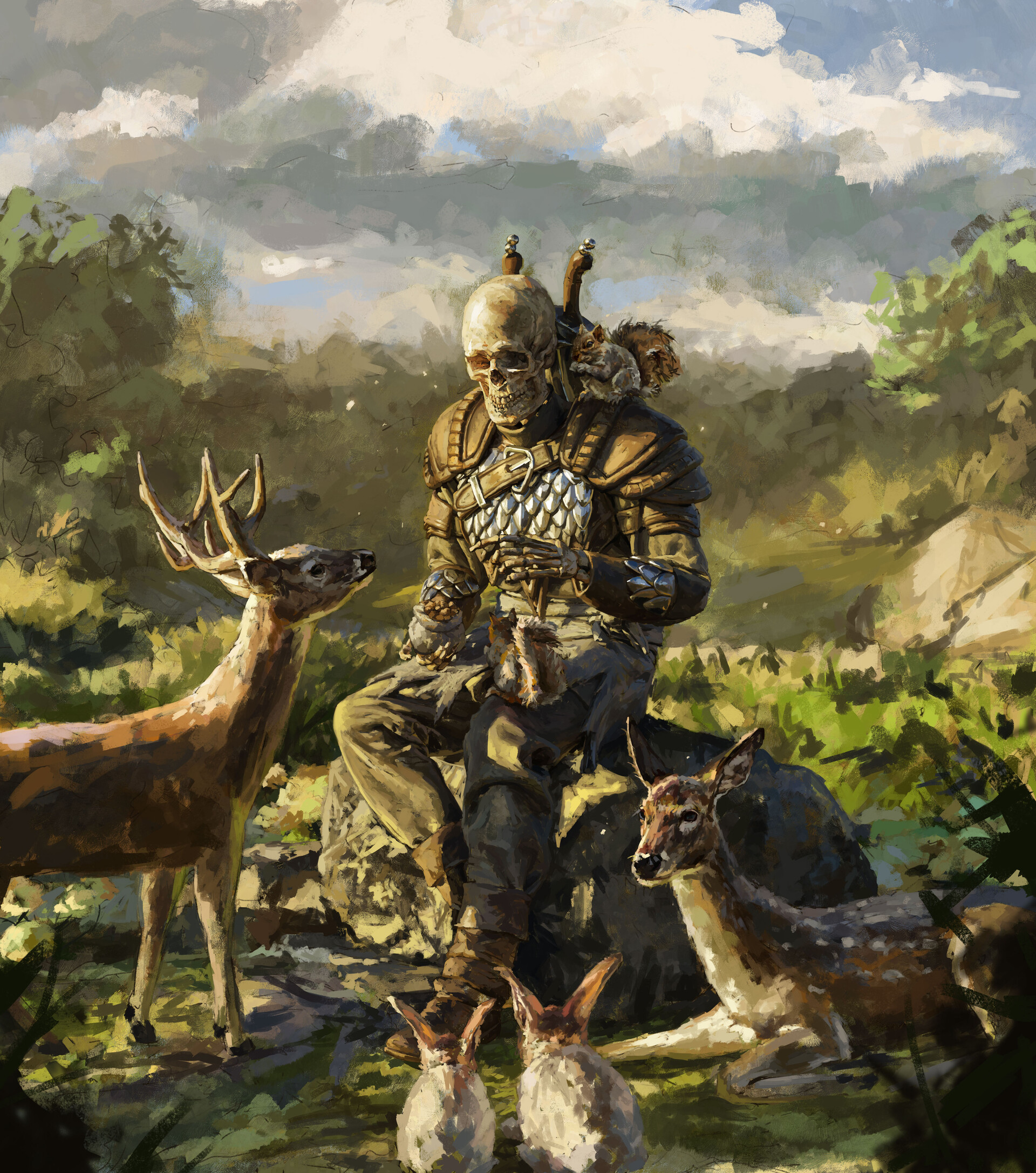In this captivating artwork, we're presented with a serene outdoor scene characterized by muted shades of green, gray, white, brown, and khaki. At the heart of the composition, a soldier with a skeleton head gazes forward while seated on a boulder. His skeletal left hand protrudes from the sleeve of his khaki or army fatigue outfit, complete with matching pants, boots, and an assortment of gear strapped to his back.

The soldier is enveloped by a rich tapestry of wildlife. To the lower left, a regal deer gazes up at him, its front legs emerging from the left side, and its antlered head turned eastward. At the soldier’s right side, a female deer, distinguished by the delicate spots adorning her back, lies peacefully on the ground. Adding a touch of whimsy, a small squirrel perches on the soldier’s left shoulder.

Nestled at the soldier’s feet, two rabbits sit side by side, their backs to the viewer. They showcase a blend of white and gray fur while their ears stand alert in an amber hue. The scene takes place in a wooded area, evidenced by patches of green interspersed with stones and rocks, under a canopy of muted trees. The background reveals a palette of greens ranging from olive and hunter to pale lime, leading up to a sky filled with gentle hues of white, gray, and light blue.

This illustration masterfully blends the eerie and the natural, creating a harmonious yet thought-provoking scene.